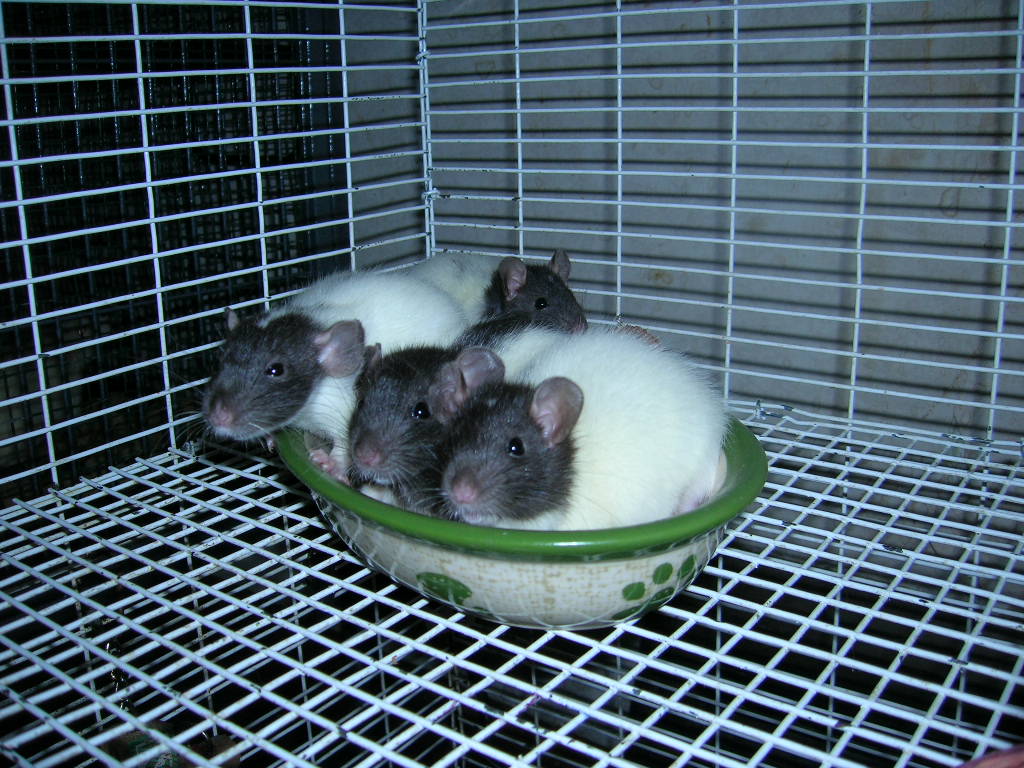This is a detailed photograph of the inside of a white metal grid-style cage. The cage's sides and floor are visible, with a white wall in the background and possibly a dark wall or door on the left. In the center of the cage sits a small bowl, cream-colored with a bright green rim and a green design resembling polka dots or a dog print. Inside this ceramic or porcelain bowl are four rodents, likely rats or mice. These animals have fluffy white bodies with black or gray fur on their heads. They possess light brown or pink round ears, dark brown beady eyes, little pink noses, and whiskers that protrude from either side of their faces. While three of these rodents face the camera, one in the back looks towards the right. All of them are huddled together in the bowl, sitting quietly and appearing to stare intently.